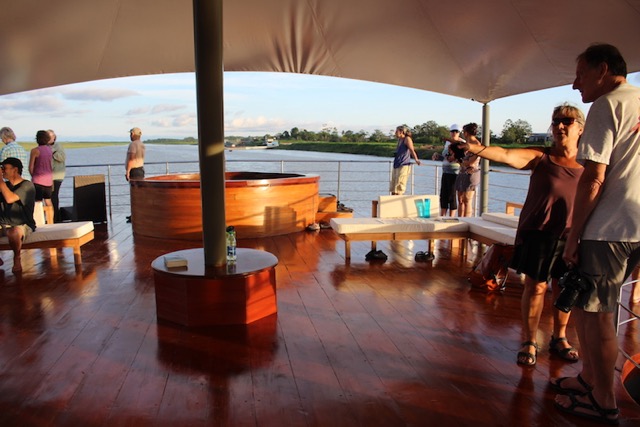A group of people are relaxing on the deck of an upscale yacht, which is likely out on the water. The deck is spacious with dark brown, shiny wooden planks. A white canopy, curved upward, provides shade for the people onboard. In the center of the deck stands a black metal pole with a circular base, supporting the canopy. At the base of the pole is a circular table with a bottle containing light yellow liquid.

On the right side of the deck, a man in a gray shirt, his head slightly tilted downward, stands next to a woman in a brown tank top and dark sunglasses. She has her arm stretched out, pointing towards the left. Toward the back left, a woman wearing a purple tank top and khaki shorts leans against the white metal barrier that lines the boat's perimeter. Further left, another person can be seen wearing a pink tank top.

A white-cushioned bench provides seating, with a man in a gray shirt sitting and gazing to the left. Near the back of the deck, there appears to be a hot tub-like structure, with wooden steps leading up to it. The water around the yacht is clear, adding to the serene ambiance, and the shore with visible trees and vegetation can be seen in the background. The overall scene suggests a casual atmosphere with individuals leisurely socializing and enjoying their surroundings.